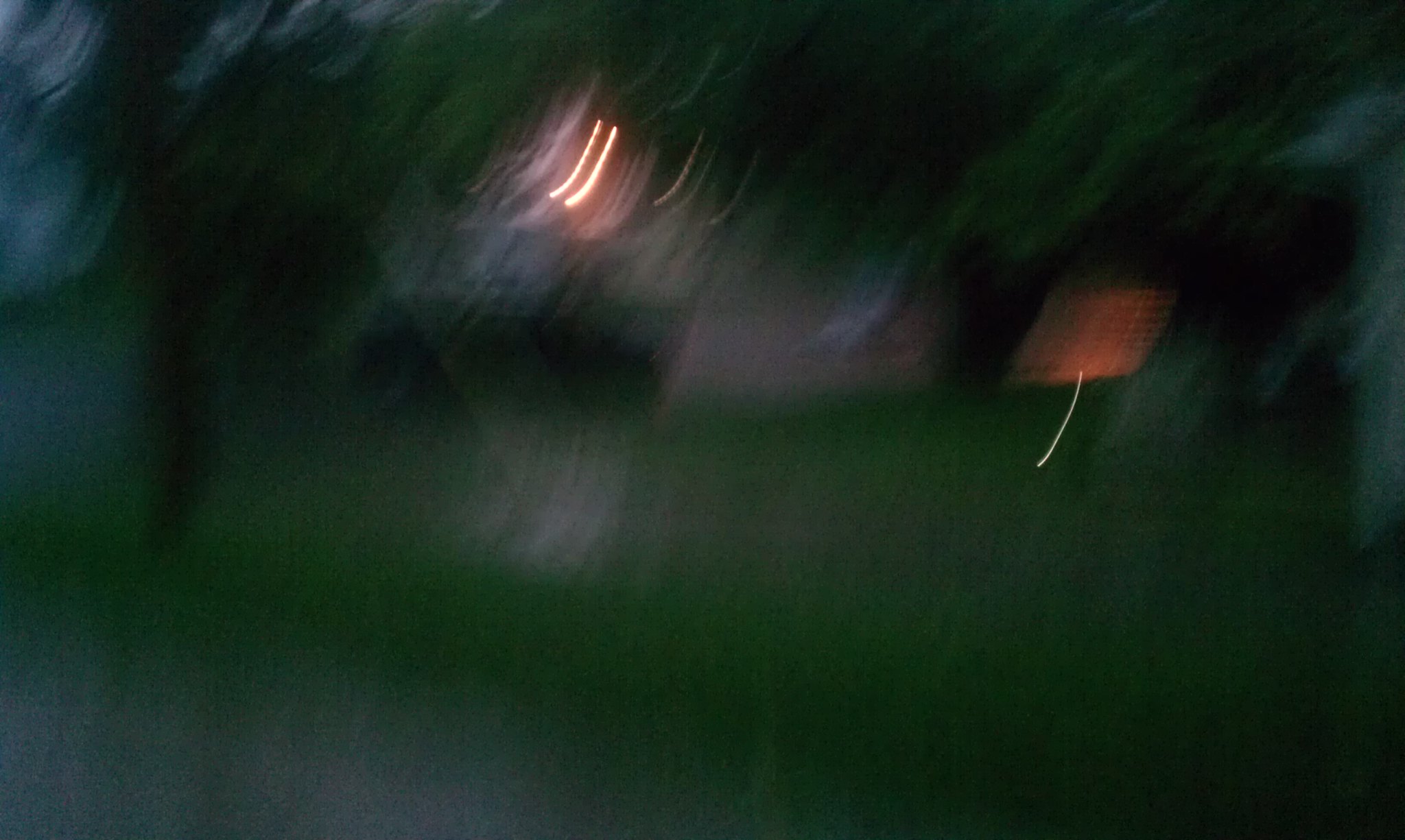This image, heavily blurred, predominantly showcases a rich green hue, suggesting a landscape teeming with foliage. The photo, seemingly captured during the early evening—approximately around 7 p.m. as the sun was in its final descent—has a dim yet discernible light quality. Amidst the blurred greenery, which hints at the presence of large trees, there is a noticeable source of light positioned in the center of the image. This illumination appears to emanate from a structure, possibly a small house or cabin, although the severe blur makes it difficult to determine the exact nature or shape of this edifice. The ambient light and surroundings imply an outdoor, rustic setting enveloped in the serenity of twilight.